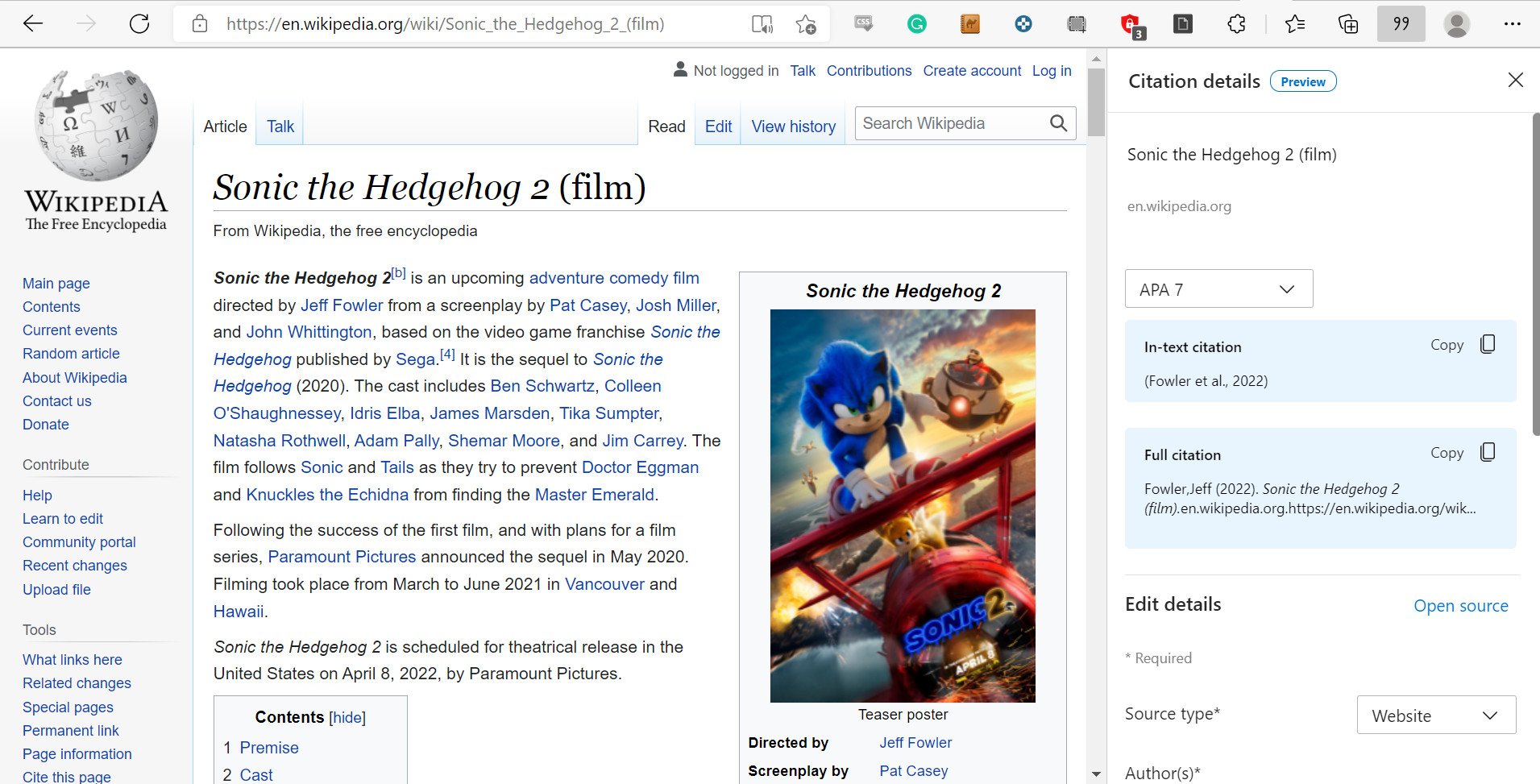The image is an informational page about Wikipedia, with the word "Wikipedia" prominently displayed in bold black text on the left side. Adjacent to this, there is an icon resembling a globe with puzzle pieces, some featuring different characters, but with its top half missing, symbolizing Wikipedia's logo.

On the right side of the page, the main header reads "Sonic the Hedgehog 2 (film)" followed by the phrase "From Wikipedia, the free encyclopedia." Below this, there is a detailed synopsis of the movie with the text color varying, including black for regular text and blue for hyperlinked entries.

Additionally, on the upper right section, "Sonic the Hedgehog 2" appears again in black text next to an image. The image depicts the character Sonic, characterized by his bright blue color, large cartoonish eyes, and distinct design. Sonic is standing on top of a vintage red airplane. Behind him, the background features fire and smoke emanating from what appears to be an enemy inside a spaceship, marked with a red dot, in pursuit of Sonic.

To the right of this image, there is a section titled "Citation Details." Inside a circle, the word "Preview" is visible. Below this, there are two blue boxes: the first marked "In-text citation" and the second, "Full citation," followed by the option to "Edit details."